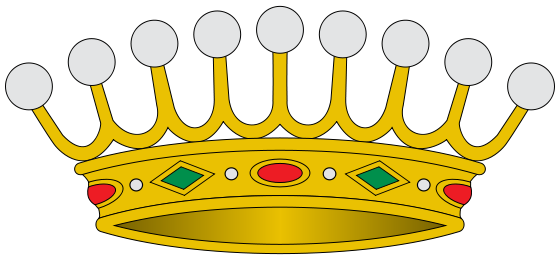This detailed cartoonish illustration features a golden king's crown floating against a plain white background in a landscape-oriented portrait. The crown's headband is adorned with a repeating pattern of gemstones: each alternating red oval gem is flanked on either side by a green rhombus, with each gem separated by a small white circle. At the top of the crown are nine large white balls, possibly representing pearls, which rest atop U-shaped gold arches. The crown's intricate design, including what appear to be rubies and emeralds, is meticulously rendered, emphasizing its grandeur and royal elegance.